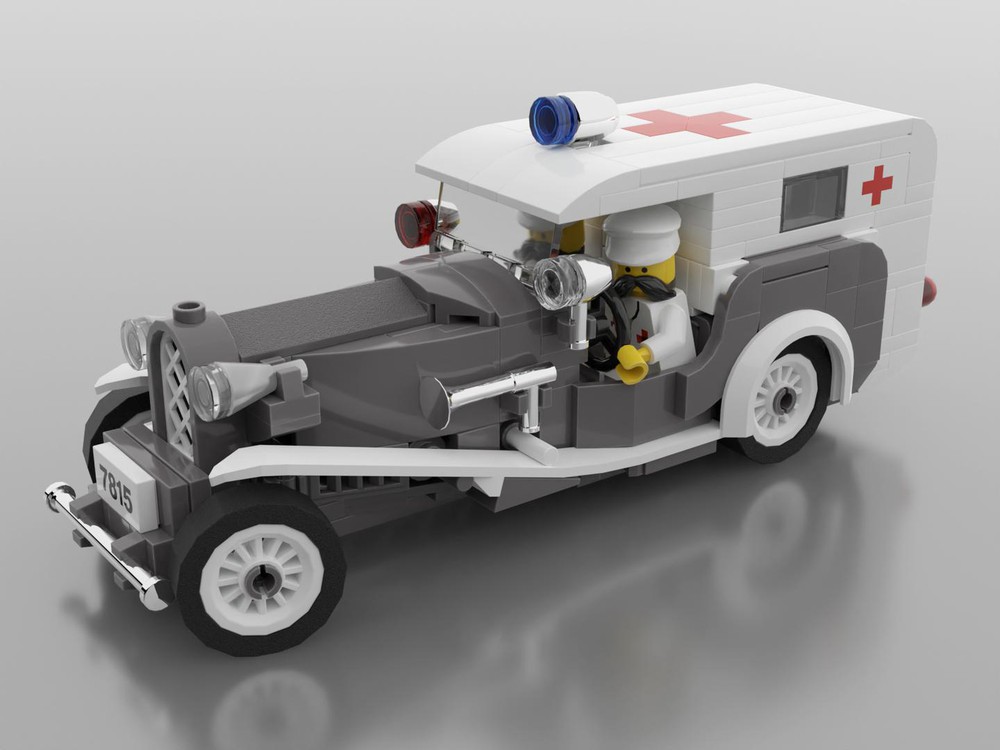The image showcases an old-fashioned, Lego-style ambulance with a blend of grey and white panels. The elongated, vintage vehicle features a white roof and back, adorned with a prominent red cross at the top and on the back right side. It includes a blue siren mounted centrally on the roof and two small lights near the windshield—one white on the left and one red on the right. The vehicle also has a chrome front bumper and a reflective grey floor beneath it. Noteworthy details include the front license plate reading "7815" and red lights on the back.

Two Lego figures with bushy mustaches and white uniforms, complete with red crosses on their chests and white hats, are driving the ambulance. Their yellow Lego hands grasp the steering wheel. This meticulously assembled or possibly 3D-rendered Lego vehicle has a significant front section, evoking a hearse or a vintage Model T car, adding to its nostalgic appearance. The entire scene is set against a plain grey background.